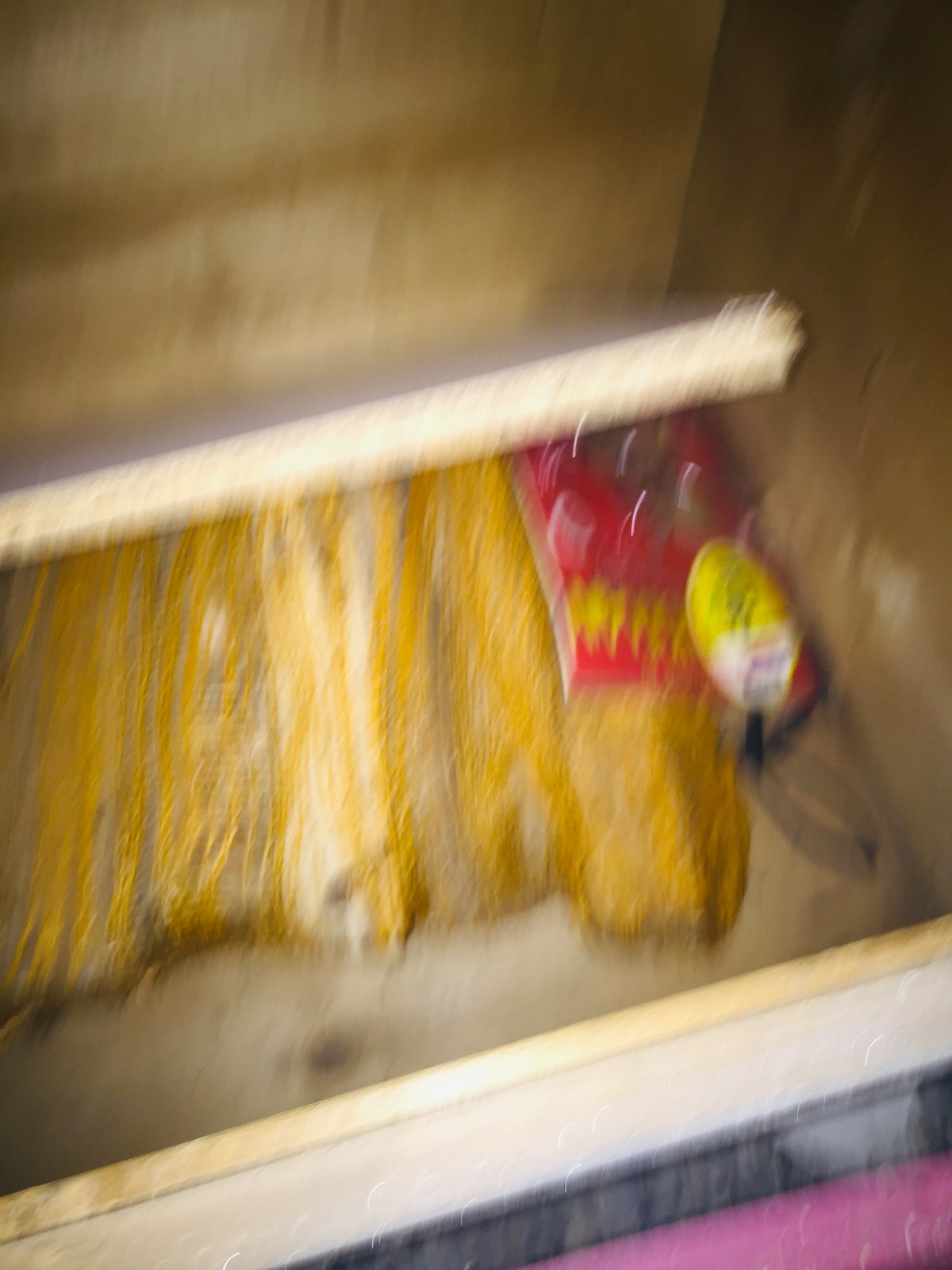This indoor blurry photograph presents a challenging view, yet certain elements are consistently discernible. The image seems to capture the contents of a wooden drawer or a small storage cabinet with the door opened upward. The wood is light in color and potentially used to store items like firewood, giving an approximate depth of five inches and dimensions about 15 inches deep and 20 inches wide. 

Inside, there are objects with tan, white, and brown portions resembling pieces of wood. Some of these objects are decorated with red and yellow markings or labels, perhaps giving an impression of a packaging or product label, which might be empty. One particularly noticeable detail is a shiny, gold material, possibly thread, in the drawer, along with a pink object in the lower right-hand corner.

At the bottom of the photo, a horizontal white-painted board can be seen, contrasting with the mauve-colored flooring visible in the bottom right-hand corner, adding to the indoor ambience.